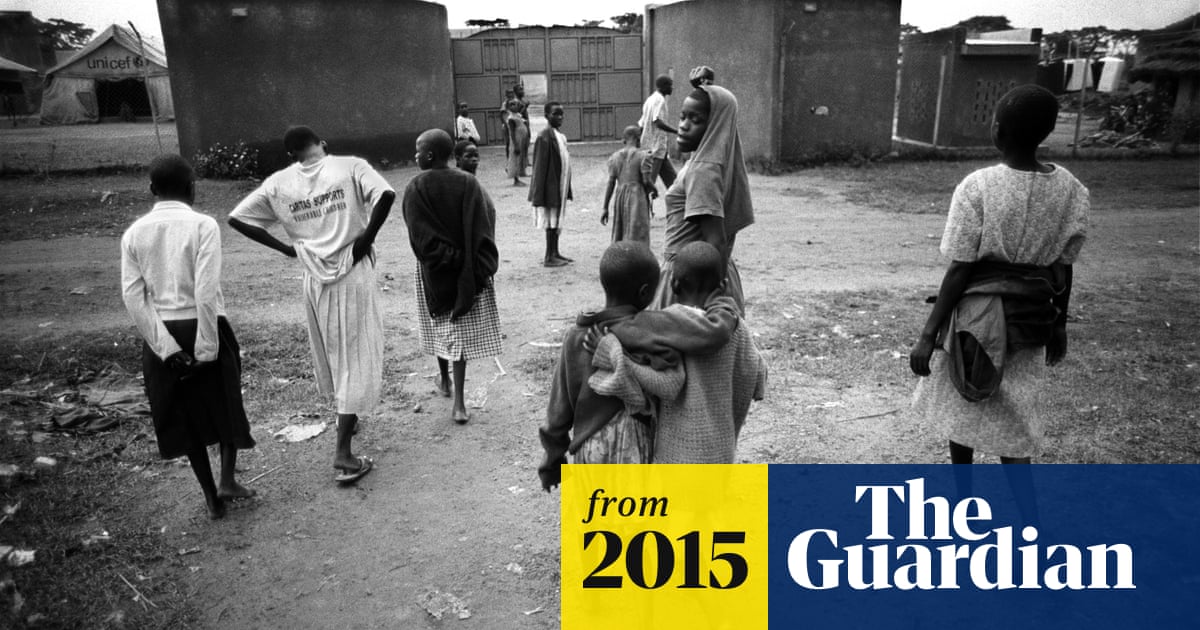This black and white photograph, titled "From 2015" by The Guardian, captures a poignant scene in what appears to be an African nation. The composition is rectangular and wide, depicting a group of African American individuals walking toward a cluster of dilapidated buildings. In the background, a structure prominently marked "UNICEF" suggests humanitarian aid in the area. The buildings, characterized by their dark tone and evident wear, resemble public housing in a distressed and impoverished setting. The foreground is littered with scattered debris, and the ground is predominantly dirt, lacking any grass. Amidst this scene, laundry hangs on lines, and two boys with arms around each other's shoulders stand out in their loose, varied clothing, which includes t-shirts, long-sleeved shirts, skirts, and dresses. The image's lower right-hand corner features a small section with color details, highlighting a yellow plaque with black font that reads "From 2015" and a blue background with white font that says "The Guardian."